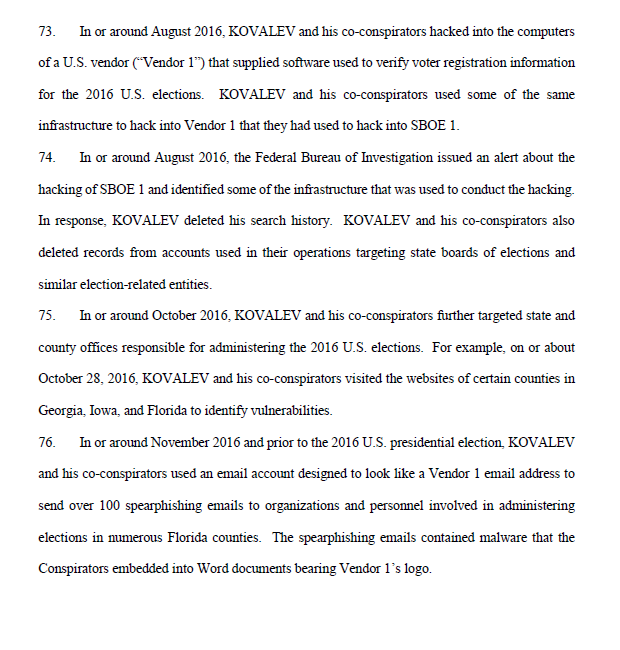The image features a plain white background with black text, likely typed on a computer. The text is formatted into paragraphs each labeled by a number, showcasing entries 73, 74, 75, and 76. Each numbered paragraph relates to a detailed account involving Kovalev and his co-conspirators' activities surrounding the 2016 United States elections. Specifically, paragraph 73 details how, in or around August 2016, Kovalev and his co-conspirators hacked into the computers of a U.S. vendor, referred to as Vendor 1, which supplied software for verifying voter registration information. It further notes that they used similar infrastructure for this hack as they had for hacking into SBOE 1. Paragraph 74 then describes how the Federal Bureau of Investigation (FBI) issued an alert in the same period about the hacking of SBOE 1, identifying some of the infrastructure used in the attack carried out by Kovalev and his team.